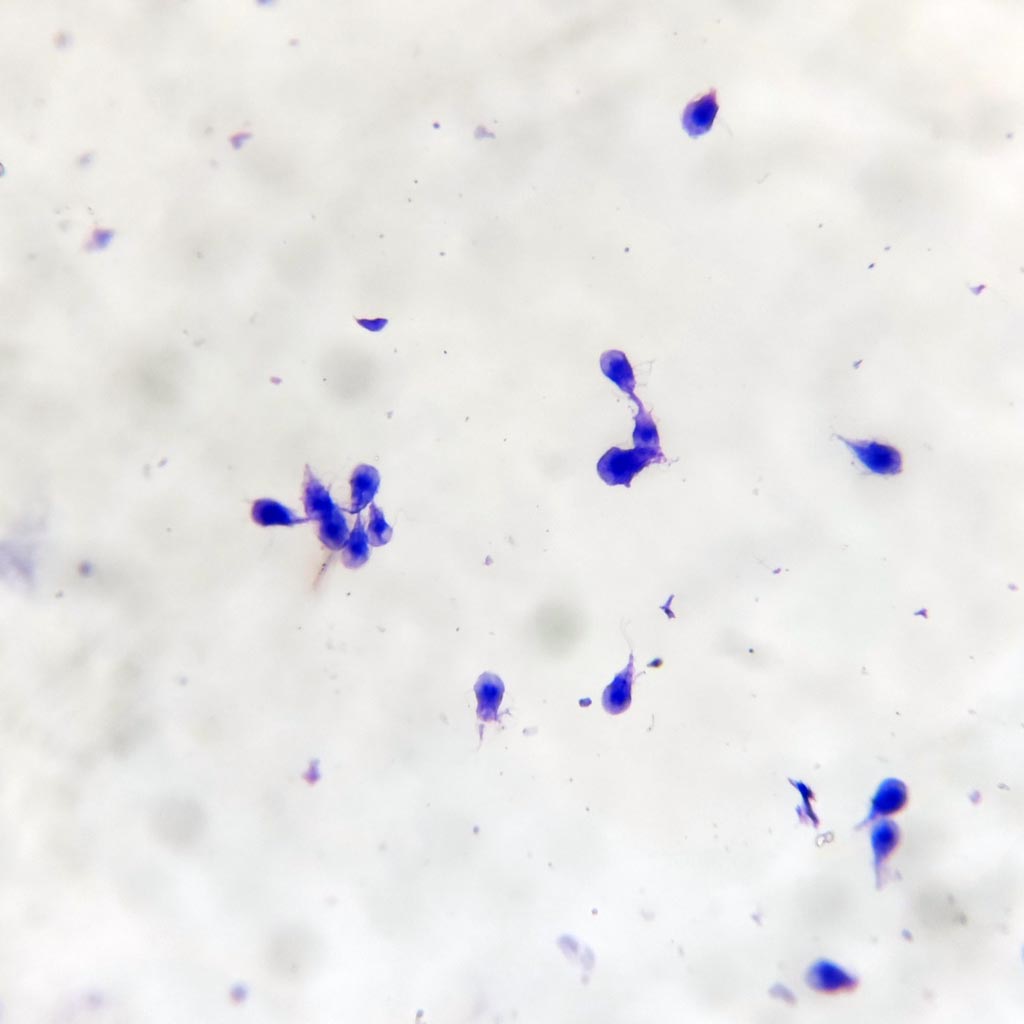The image showcases a richly detailed, deep purple splattering that appears to be on a glass surface, though it may also resemble a view through a microscope. This splattering gives the illusion that the glass reveals hidden images below, yet those images do not seem to be part of the picture itself. The paint forms various small groups and individual specks all over the gray background, with the darkest and most prominent elements on the surface.

Upon closer inspection, these purple splatters exhibit a resemblance to tiny microorganisms or single-celled organisms, each with translucent edges and darker inner parts that could be likened to organs. Some of these elements appear clustered, with groups of six or three, and others lie scattered individually, floating within what seems like a fluid medium. The background’s blotchy mix of white, pinkish-blue, and gray shades further enhances this quasi-microscopic view. Accompanying these central elements are various smaller debris and particles of the same purplish hue, giving the entire composition a sense of chaotic beauty, whether interpreted as floral petals in suspension or microscopic life forms.